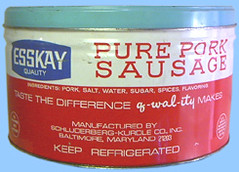The image depicts a can of sausage, characterized by its wide, cylindrical shape. At the bottom of the can, the text "Keep Refrigerated" is prominently displayed. Above this, the can's manufacturer is listed as "Golderberg, KURCLECO, Inc., Baltimore, Maryland," followed by a zip code. Near the middle of the can, the phrase "Taste the Difference" is written in cursive white text, followed by the word "makes." The ingredients are listed above this phrase and include pork, salt, water, sugar, spices, and flavoring, all set against a red background with white text. Above the ingredients section, a white background with red text proclaims "Pure Pork Sausage." To the left side of this text, a blue background showcases the words "S-K Quality" in white text. The can features a light blue colored cap, and the majority of the background behind the text and logos is also light blue.